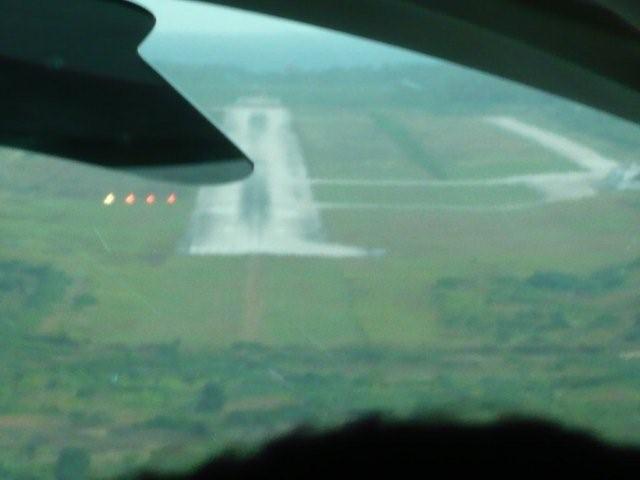This image appears to be taken from inside an aircraft cockpit, capturing an aerial view of an airfield below. The cockpit's interior structure is visible, with parts of the frame or material looming in the upper left and around the edges, featuring beige or white hues. The airfield below features extensive grassy areas interspersed with dirt, with much of the grass appearing light green, though tinged by some darker patches.

At the center of the image lies a long, prominent runway in a mix of white and dark gray tones, lined on the left side with a series of three red lights and a yellow light. Two additional square sections surround the runway on its right, resembling concrete or perhaps tarmac surfaces. The airstrip further extends into a network of smaller paths leading out to a white road positioned in the upper right.

The backdrop is faintly blurred and somewhat foggy, suggesting limited visibility or a lower quality image. There are also dark trees and bushes around the airfield, contributing to the natural landscape. The overall composition suggests a daytime scene, possibly indicating early morning or hazy weather conditions that diffuse the light across the field.